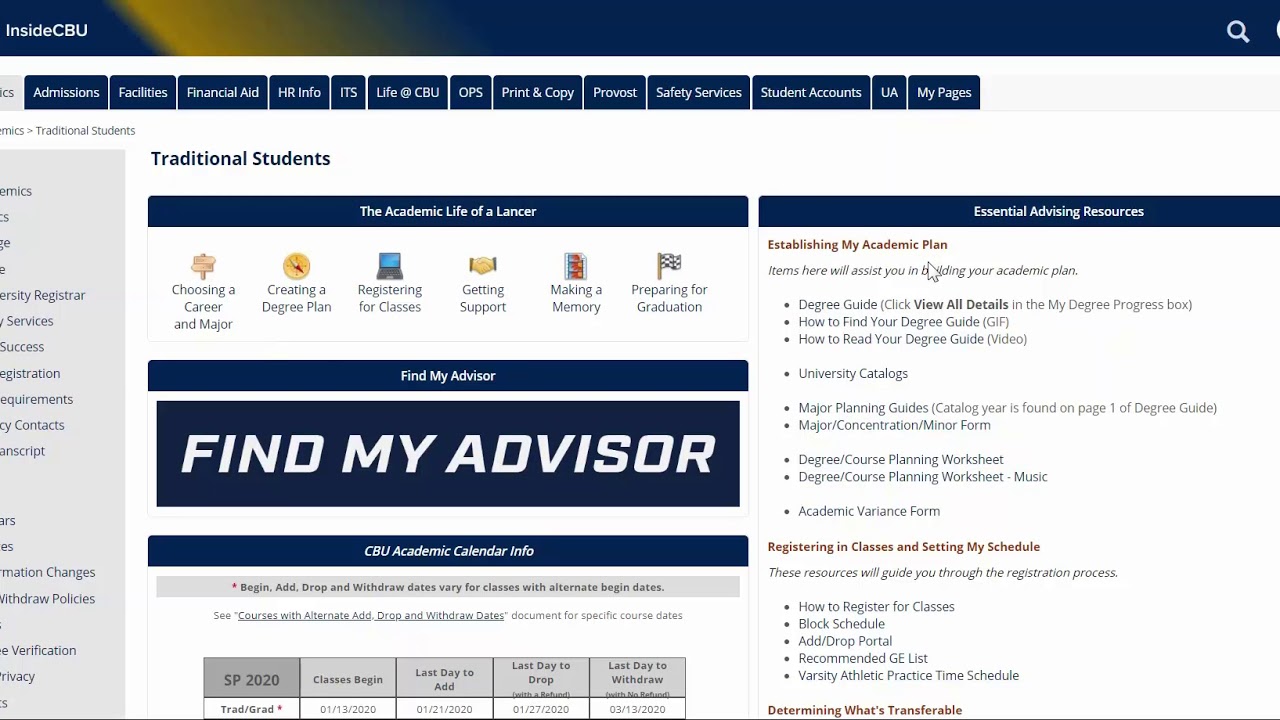The page belongs to a website titled "InsightCBU" at the top, suggesting it's part of a portal for California Baptist University. To the right at the top, there's a search function. Below, there are numerous navigation tabs—approximately 12 to 14—with a blue background and white text. These tabs are labeled as Admissions, Financial Aid, HR Info, ITS, Life at CBU, OPS, Print and Copy, Provost, Safety Services, Student Accounts, UA, and My Pages. The currently selected tab is cut off in the image.

On the left side, there's a gray sidebar containing sections for contact information and verification, though the text is partially cut off.

The main content section in the center-right focuses on traditional student resources under "The Academic Life of a Lancer." Key buttons include Choosing a Career and Major, Creating a Degree Plan, Registering for Classes, Getting Support, Making a Memory Plan for Graduation, and Finding My Advisor—this section is prominently highlighted. Additional resources listed include the CBU Academic Calendar, Scheduling Classes, Essential Advising Resources, Establishing an Academic Plan, Degree Guide, University Catalog, Registering Classes, and Information on Transfer Credits.